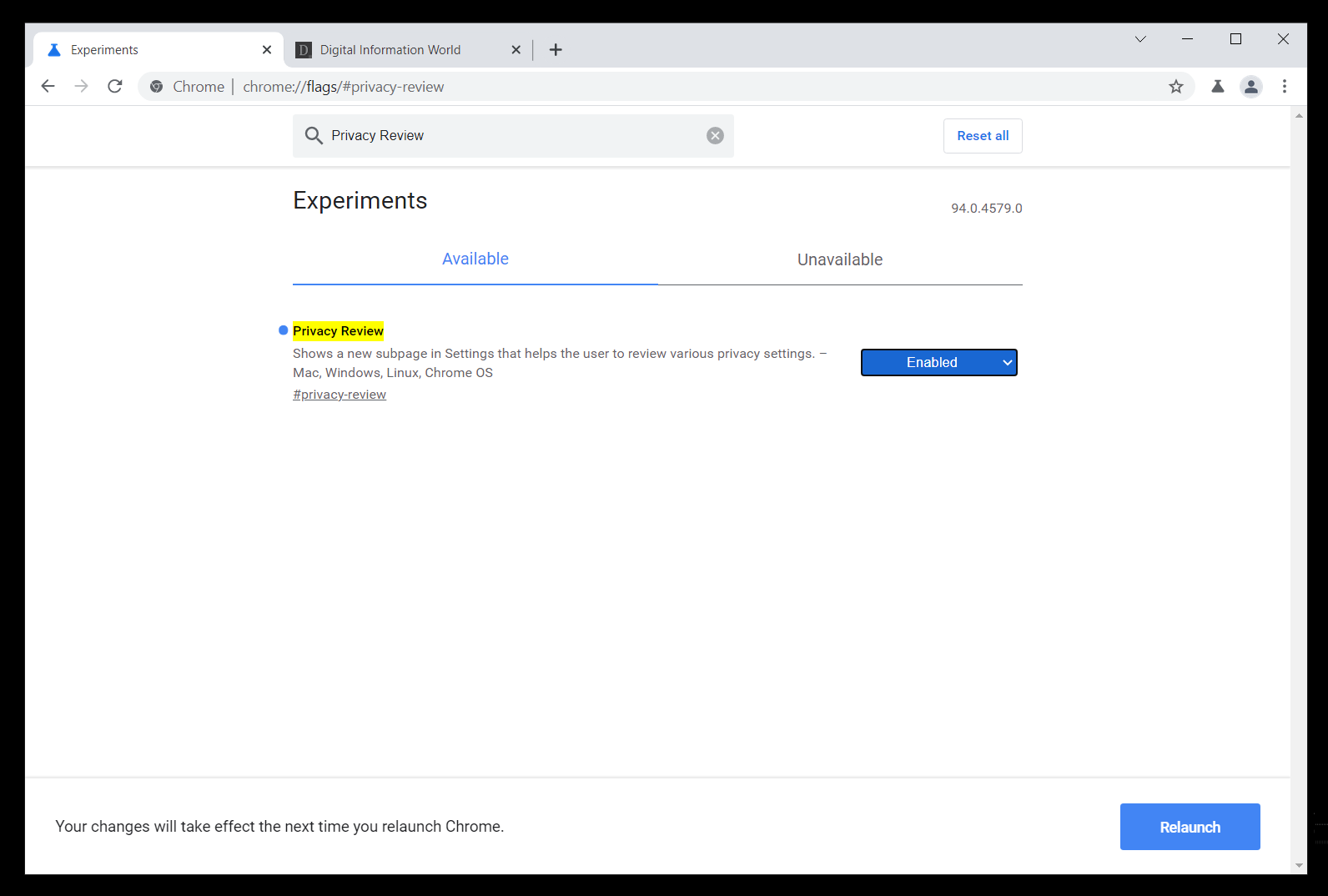The image displays a section of a website titled "Experiments." At the top right corner, there are two browser tabs. The white tab, marked "Experiments," features a blue icon, while the gray tab, labeled "Digital Information World," bears a black icon.

Below the tabs, the page content begins with references to "Chrome," "Chrome Flags," and "Privacy Review." A gray search bar labeled "Privacy Review" includes a search icon and a "Reset All" option in blue, set against a gray background.

Prominently positioned in large black letters is the heading "Experiments," accompanied by sections labeled "Available" and "Unavailable." The "Available" section is highlighted in blue, with a blue bar beneath it. Adjacent to the "Experiments" heading, some numerical indicators are visible.

Under the "Available" section, the "Privacy Review" title appears with a blue dot next to it, highlighted in yellow. It includes the description: "Show a New Subpage and Settings that helps the user to review various privacy settings. Mac, Windows, Linux, Chrome OS." Following this, the term "Privacy Review" is reiterated.

On the right side of this section, a blue box with white text that reads "Enabled" is visible, accompanied by a dropdown arrow.

At the bottom of the image, a message states, "Your changes will take effect the next time you relaunch Chrome." Below this message, a blue button with white text labeled "Relaunch" is present.